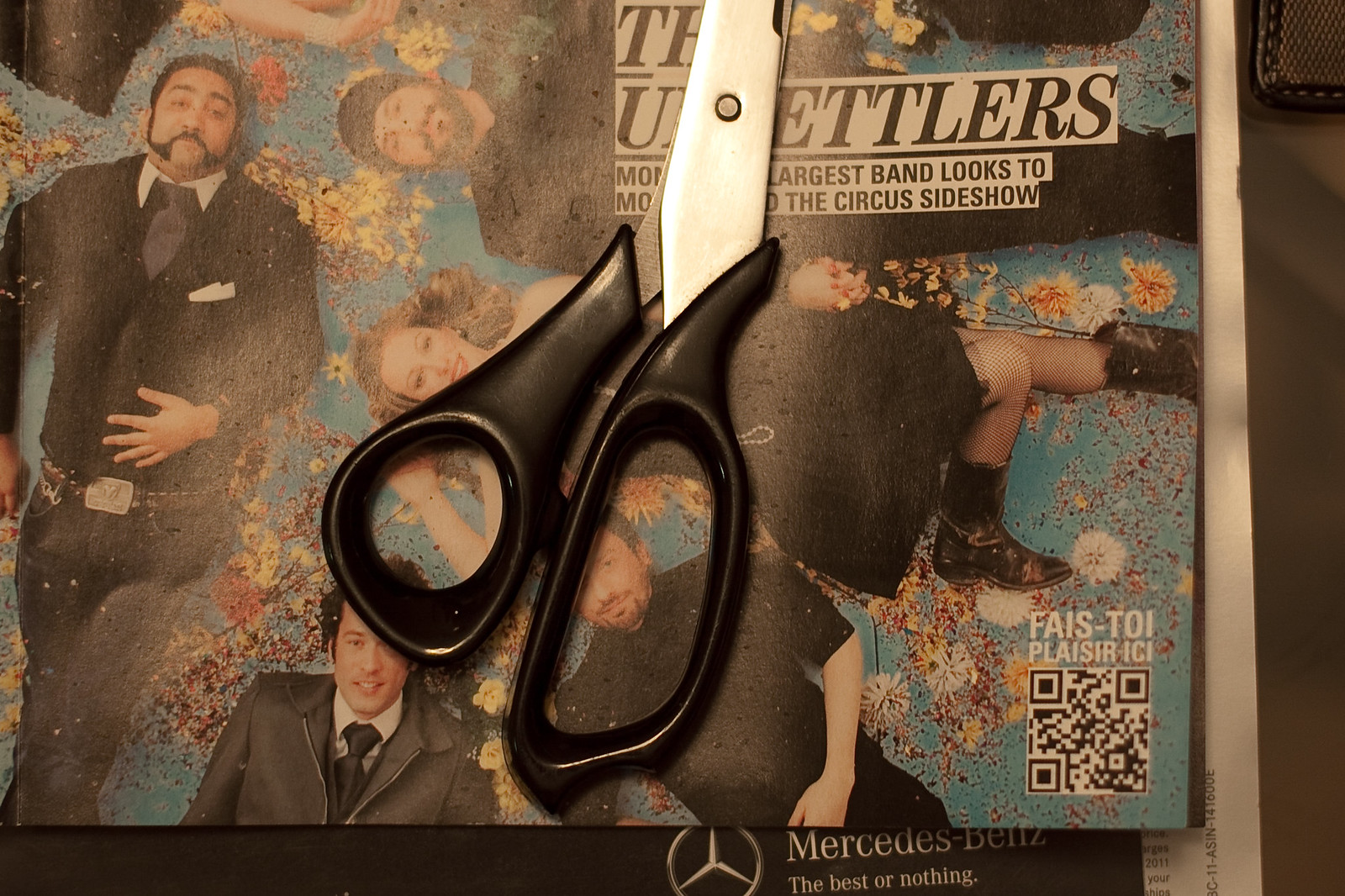In the center of this image is a pair of black-handled scissors with silver blades, which immediately draw attention. The scissors rest on top of magazine pages featuring a band. The band members are arranged in a loosely circular, interspersed pattern, seemingly laying on the ground. The man on the left sports an old-timey goatee connecting to his mustache, wearing a sophisticated black outfit with a white pocket square, tie, and a fancy belt. Below him, another man in a silvery zip-up jacket and tie smiles at the camera. To the right, a gentleman in a black short-sleeved shirt with scruffy facial hair accompanies them. A woman with light brown honey-blonde hair lies horizontally, dressed in a black dress, fishnet tights, and black boots. Beside her, a man in a black beanie with a full beard also wears all black. 

The magazine cover partially reveals the band's name, which seems to begin with "THE" and includes the letters "U" and ends in "ETLERS," suggesting it may be "THE SETTLERS" or a similar name. The headline teases "largest band looks to MO," with the remaining text obscured by the scissors. In the bottom right corner, a QR code and French text "FAIS-TOI PLAISIR ICI" juxtapose with a Mercedes-Benz logo and the slogan "The best or nothing." A detailed setting including a dark brown background off to the right, black leather edging with white stitching, and some greyish brown fabric completes the visual context, hinting at an artsy, scrapbook-like composition.